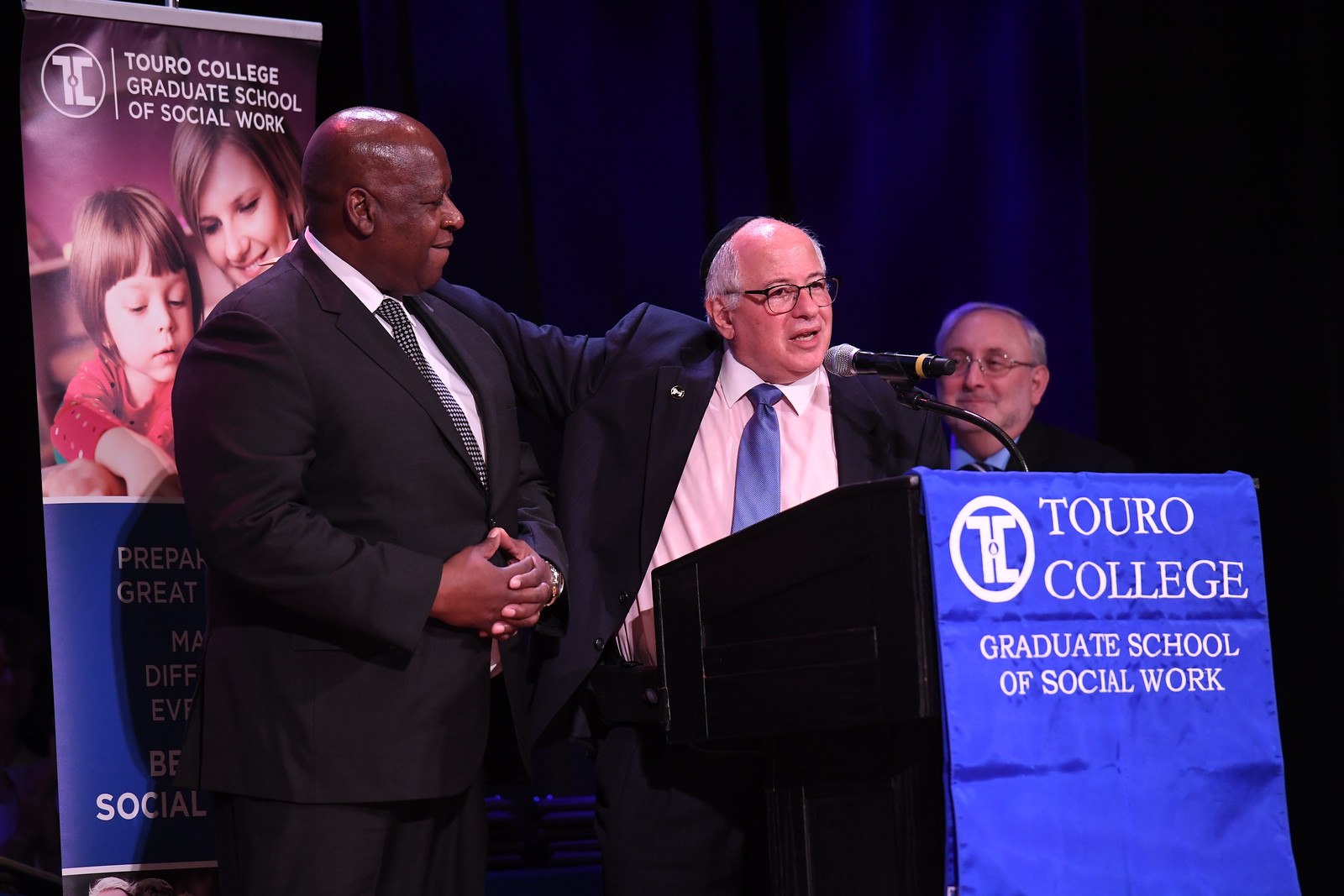The image captures a significant moment at an event likely held at Touro College's Graduate School of Social Work. Three men, dressed in similar gray suits, are on stage. The central figure, an older Caucasian man in his 60s with balding gray hair and glasses, appears to be delivering a speech at the podium, which prominently displays the Touro College Graduate School of Social Work insignia in bright blue and white.

Standing closely to his right, with a supportive arm around his shoulder, is a tall, heavy-set African man who is smiling, perhaps being acknowledged or receiving an award. His fingers are crossed in front of him, indicating his pleasure and anticipation of the speech. In the background, a shorter Caucasian man with a full head of gray hair and glasses is seated on stage, observing the scene.

The backdrop features a bold banner with the Touro College Graduate School of Social Work logo, including an image of a mother and child, symbolizing the school's focus on social work. A blue curtain drapes behind them, adding a formal touch to the event setting.